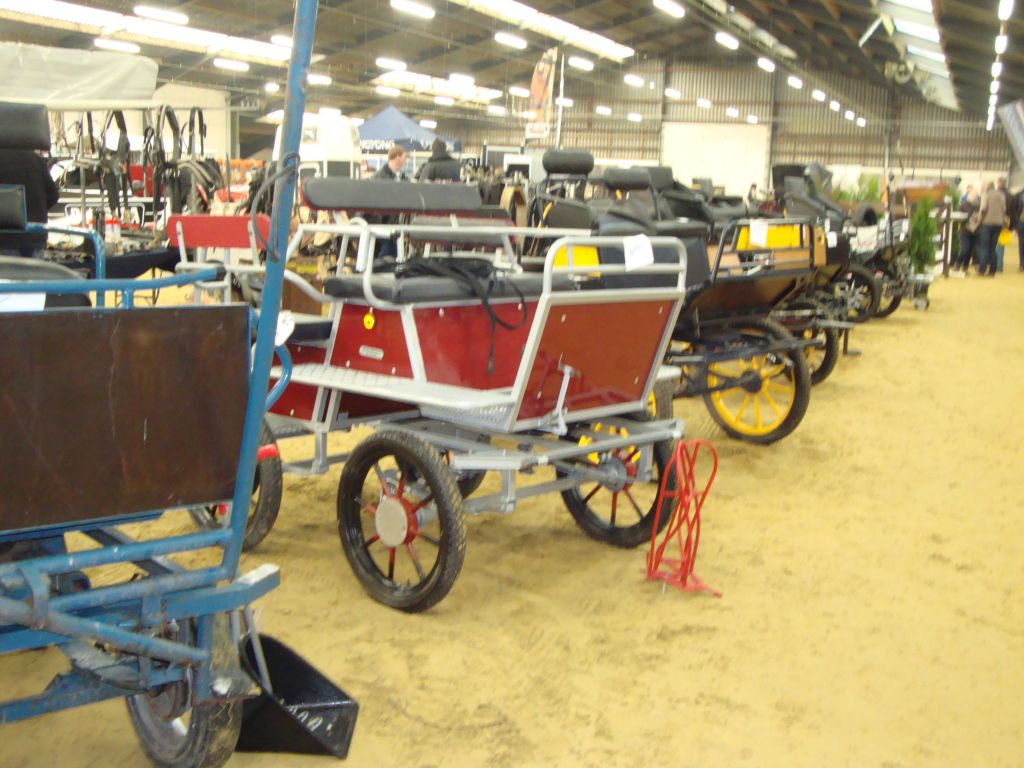This photograph captures the interior of a large warehouse or pole barn, resembling a fairground building, illuminated by numerous hanging lights. The ground is a beige, tan-brown color, possibly dirt or sand. The main focus of the image is a collection of horse-drawn carriages or buggies lined up in a row, each varying in shape, size, and color. The nearest buggy is a vivid blue and has one visible wheel. Prominently displayed in the center of the image is a red buggy with all four wheels visible and ropes for horse attachment, lacking any overhead cover. To the left, there are additional buggies, including a black one and another that appears to be covered. In the background, some harnesses and tents can be seen. Various people are scattered throughout the space, with a group of three or four individuals talking to each other on the far right. Above the red buggy, two more people are visible but not facing the camera.